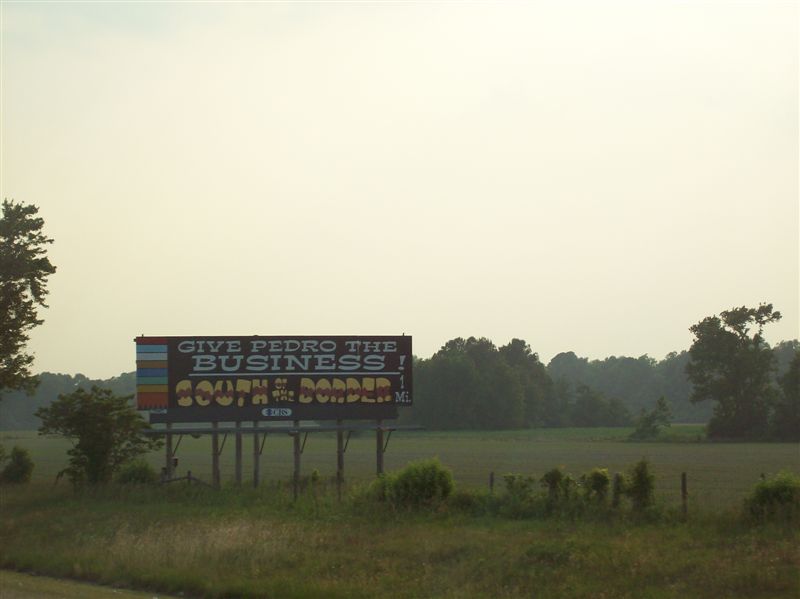This photograph captures a striking billboard situated in a rural field. The billboard itself is black, adorned with bold white lettering that reads, "Give Pedro the Business." Beneath this phrase, in a yellow and brown font, is the phrase "South of the Border." This suggests that the billboard is advertising a small business or tourist attraction. 

The landscape surrounding the billboard features sparse, short vegetation, indicative of a field. In the background, a row of trees frames the scene, emphasizing the billboard's prominence. At the lower left corner of the image, what appears to be a dirt road—a light brown path—stretches out, suggesting rustic accessibility. Adding to the rural charm, a wooden fence with barbed wire borders the field, reinforcing the rustic and remote atmosphere.

The overall scene is under a blanket of overcast, cloudy skies, lending a soft, diffused light to the entire image. This weather condition enhances the simplicity and quietude of the setting.